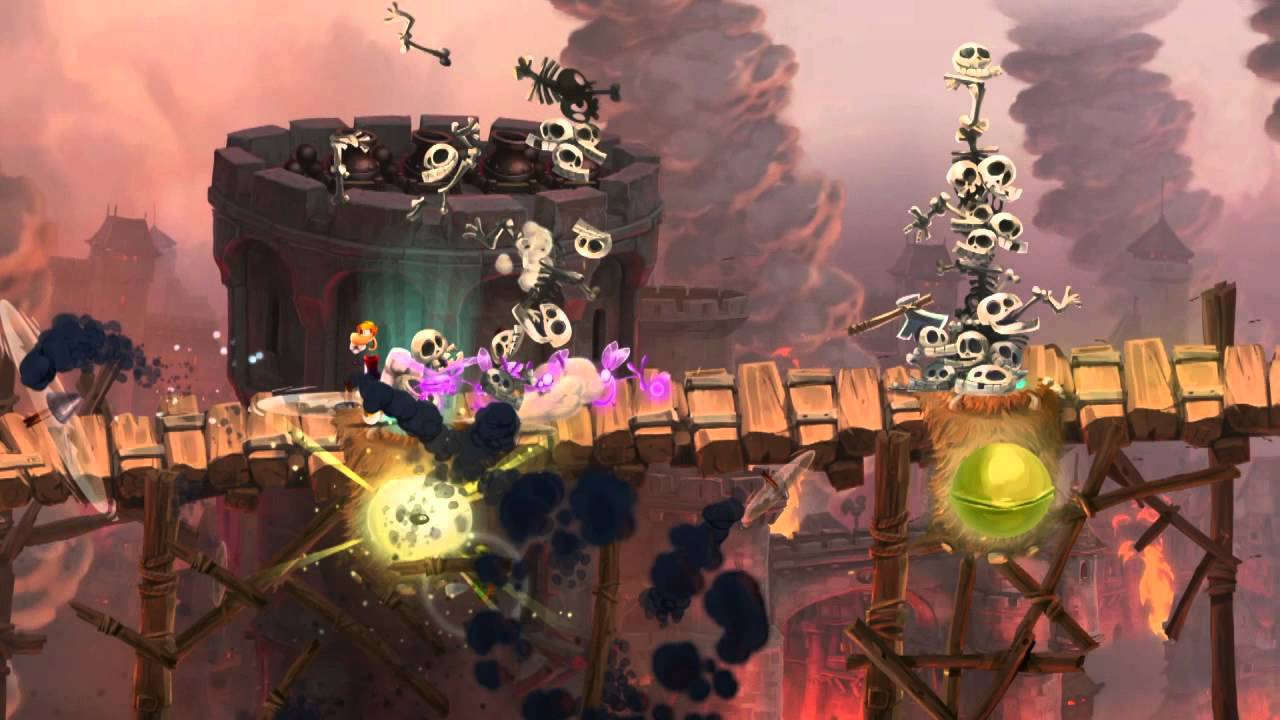This detailed illustration appears to be a scene from a painting or possibly a video game. It features a wooden bridge strewn with skeleton remains and human skulls. On the right side of the bridge, there is a meticulously stacked tower of bones, primarily human skulls, held together by other skeletal pieces. Directly opposite, on the left side, the structured pile of skulls is depicted mid-destruction, as if it were hit by a catastrophic explosion, with skulls violently scattering through the air. An explosion seems to be triggering this chaos from beneath the bridge.

The background is dominated by thick clouds of black smoke rising into an amber-hued sky, creating an ambiance of war and destruction. A castle in flames looms beyond this chaotic foreground, with sections of it faintly visible amidst the smoke on the left side of the bridge. The painting's color palette includes hues of pale pink, pinkish-gray, brown, and yellow, with notable white skulls and yellow orbs that might represent bells placed at the base of the skull piles, also caught in the explosion on the left side.

Overall, the image intricately combines elements of destruction and decay set against the eerie, smoldering backdrop of a burning castle.